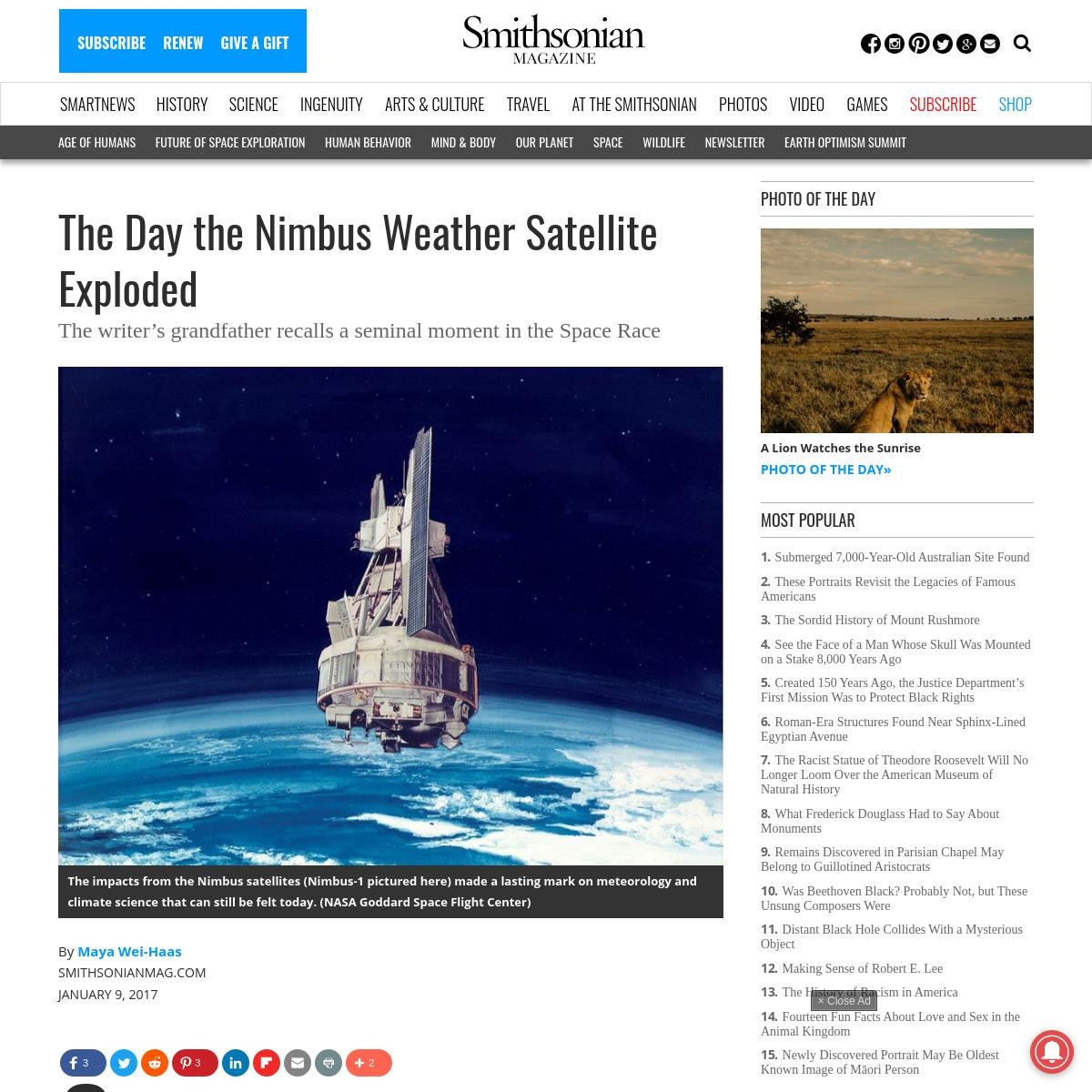Screenshot of the Smithsonian Magazine website. At the top center, the "Smithsonian Magazine" logo is prominently displayed. To the left, blue buttons offer options for "Subscribe," "Renew," and "Give a Gift." The top right corner features icons and links to social media platforms such as Facebook and Twitter.

Below the header is a navigation bar with tabs labeled "Smart News," "History," "Science," "Ingenuity," "Arts & Culture," "Travel at the Smithsonian," "Photos," "Video," "Games," "Subscribe," and "Shop." Directly beneath these tabs are additional clickable options including "Age of Humans," "Future of Space Exploration," "Human Behavior," "Mind and Body," "Our Planet," "Space," "Wildlife," "Newsletter," "Earth Optimism," and "Submit."

On the right side of the page is a column titled "Photo of the Day," displaying an image of a lion in the safari. The caption reads, "A lion watches the sunrise." Below this column is a list of the most popular articles from Smithsonian Magazine.

Dominating the left side, the main article is titled "The Day the Nimbus Weather Satellite Exploded." The subtext explains, "The writer's grandfather recalls a seminal moment in the space race." Accompanying the article is a large image of a spacecraft floating above Earth. The image caption states, "The impacts from the Nimbus satellites, Nimbus 1 pictured here, made a lasting mark on meteorology and climate science that can still be felt today." Credit is given to NASA Goddard Space Flight Center. The article is authored by Maya Weihai and was published on January 9th, 2017.